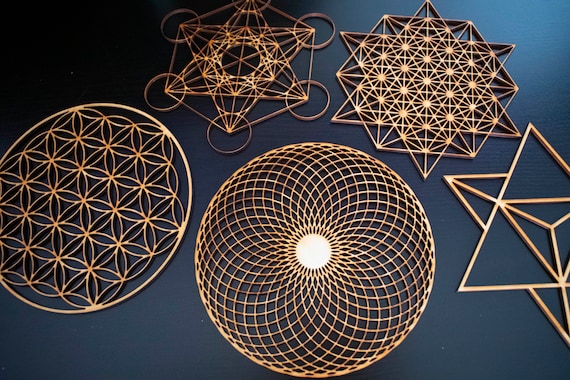In this striking image set against a blue background, intricate sacred geometry patterns made from a copper-like, golden metal are showcased in stunning detail. The geometric designs, shimmering under a light source that highlights their metallic sheen, create a harmonious blend of art and mathematics.

At the bottom center, multiple interlocking circles form a complex diamond pattern, converging at a radiant golden center. To the right of this central piece is an outline resembling a star, while to the left, floral-like shapes meld into a circular formation. The top left features a Metatron's Cube, with six circles punctuating the points of the pattern, closely resembling a detailed pentagram. Adjacent to it is an ornate shape composed of interconnecting triangles, with gold dots marking their intersecting points.

The entire composition presents hollow designs, allowing the blue background to peek through, emphasizing the complexity and beauty of the golden sacred geometry patterns. Each pattern, meticulously crafted, contributes to a mesmerizing tableau that blends mysticism and art in a visually spectacular manner.